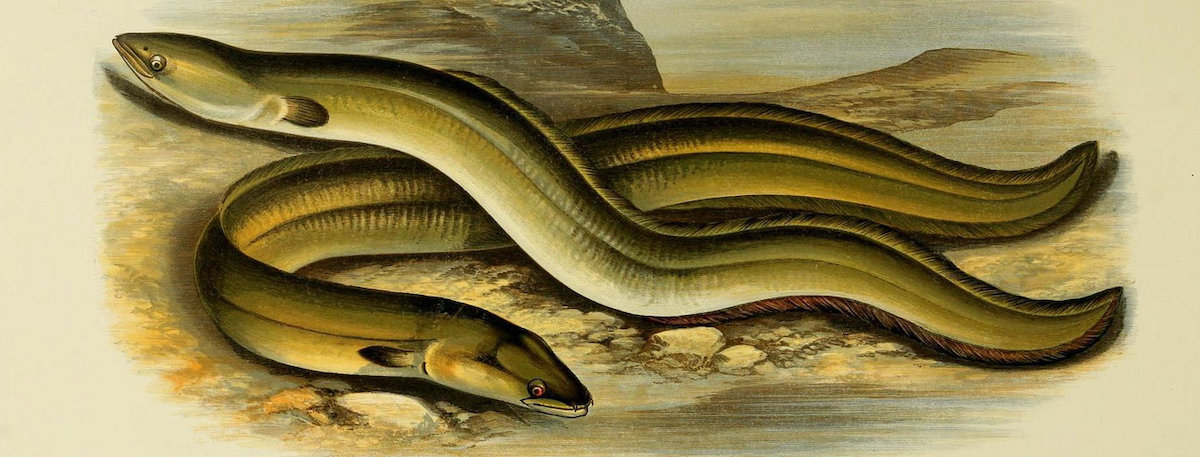The image appears to be a sophisticated lithograph painting of two eels, evocative of an older 20th-century artwork. These eels, which could be mistaken for snakes due to their elongated, wavy forms, are depicted with impressive detail. Their bodies are predominantly greenish-yellow with brown and orange highlights, creating a rich, somewhat iridescent color palette.

Both eels are shown against a backdrop of yellowish-gray stones, suggestive of a riverbank or a sea bottom. The eel on the bottom is curled back with its head pointing towards the center, while the one on top faces towards the top left side of the painting. Small, hair-like fibers and fins are noticeable along their bodies, hinting at the possibility that these eels might represent an extinct species.

The background is characterized by a hazy blue sky, blending seamlessly into the indistinct, white-bordered edges of the scene. This careful composition and color blending create a visually complex and detailed representation of these aquatic creatures, capturing an underwater or riverside setting.